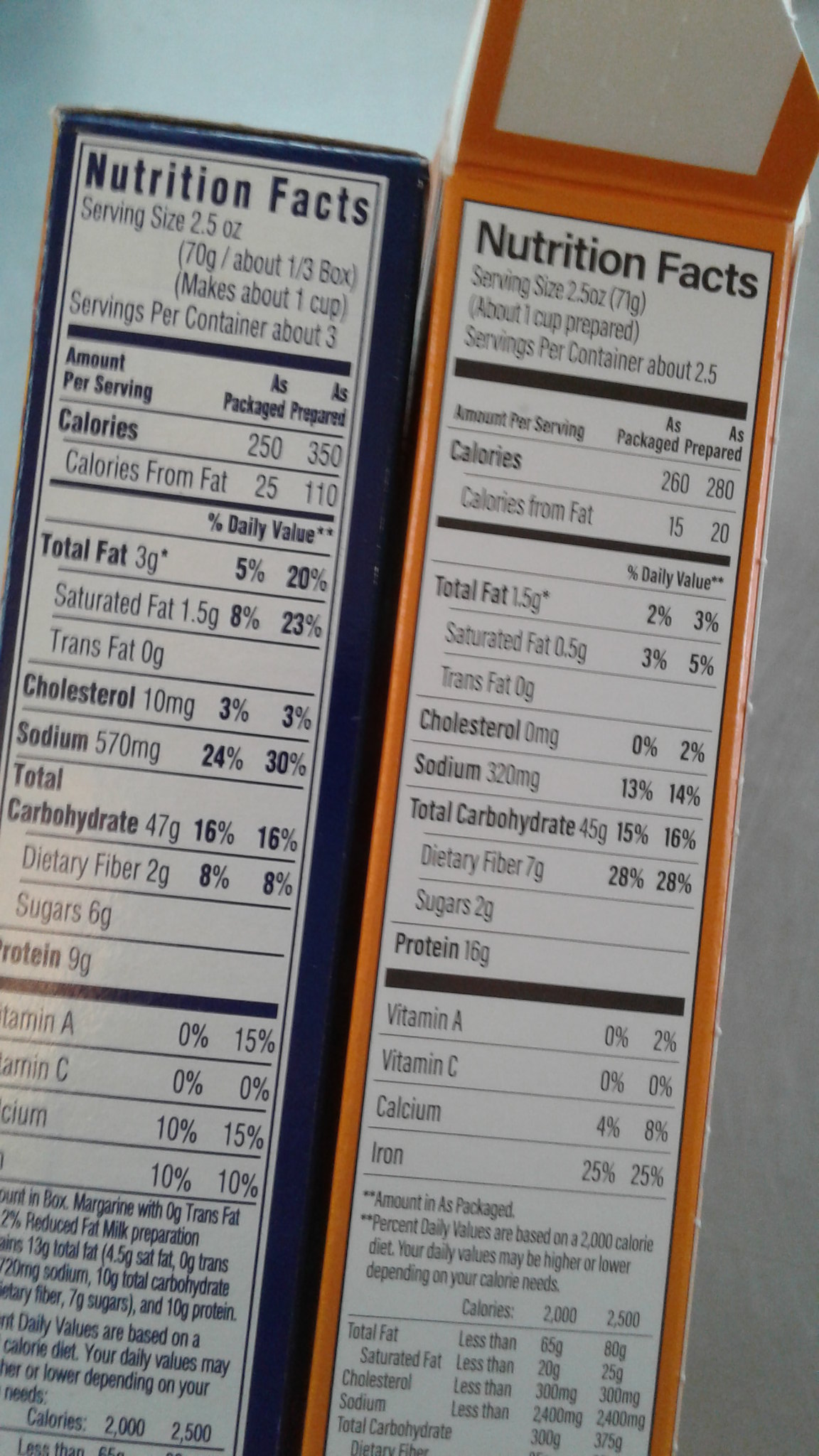The photograph showcases two boxes placed side by side on a slightly textured white surface. The left box is a deep navy blue with a prominently displayed white label featuring navy-colored font. The right box is a vibrant orange, also adorned with a white label but in contrasting black font. Both labels are meticulously detailed, highlighting nutritional information such as serving size, calories, fat content, and saturated fat levels. The navy box’s ingredient list is partially visible, while the orange box’s nutrition label is exceptionally comprehensive. Light gently reflects off the nutrition label of the navy box, adding a touch of dimension to the scene.